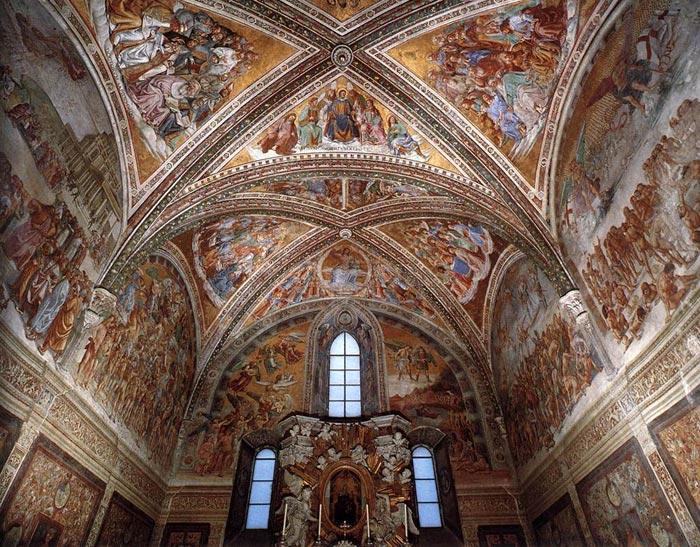The image captures the intricate and expansive interior of what appears to be an old-fashioned church or cathedral, likely boasting a ceiling that reaches 100 feet or more in height. The photograph prominently displays a ceiling adorned with elaborate murals, divided by intricate architecture. These murals depict various religious scenes, including images of Jesus, angels with wings, cherubs, and numerous figures thought to be his disciples, local women, and worshippers.

At the center of the chapel, there are three arched windows—one positioned at the top, with the other two on the left and right sides. Underneath these windows resides a magnificent gold altar-like structure, surrounded by statues of angels. In front of the altar, there are four white pillar candles, and at the very base of the altar stands a small gold cross.

The detailed murals on the walls and ceiling contribute to the grandeur of the space, evoking Renaissance art with their vivid portrayal of holy figures, including the wise men in varied colored robes. Throughout the ceilings and walls, groups of individuals are depicted in various tableaux, some appearing to engage in daily life or walking around architectural elements, while others are shown in scenes that illustrate pivotal moments in religious narratives. Some figures are depicted unclad, adding to the complexity and depth of the artwork.